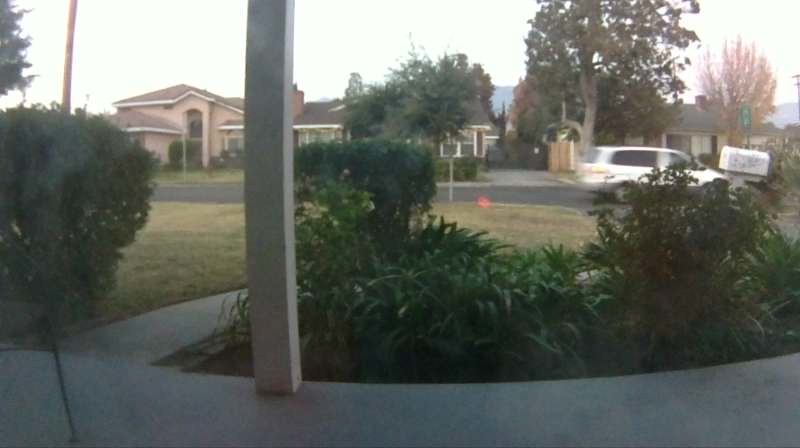The outdoor photograph captures a daytime view from a concrete-floored porch, looking out into a front yard and extending into a two-lane street in the distance. Prominently, a white, square support post stands left of center in the foreground. The porch is bordered by lush, green shrubbery that partially obscures a white van moving from left to right on the street. The yard shows a freshly mowed grass lawn intersected by a diagonal concrete path, partially hidden by the landscaping at the edge of the porch. Dominating the left background is a large brown or tan single-story house, while a cluster of trees and a partial profile of a white or gray mailbox occupy the right background. Additionally, a brown utility pole can be seen to the left, though the overall image remains slightly hazy and out of focus, despite being well lit.